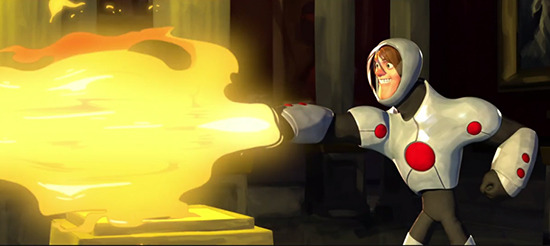In this detailed scene from a 3D kids' animation, a character clad in a sleek silver-white armor stands amidst a dark forest. The armor is accentuated with red dots and features robust gauntlets. The character, a white man with brown hair, wears a silver helmet with a clear face shield, and he is smiling broadly, visibly thrilled by his actions. His right arm, equipped with a flamethrower-like mechanism, emits bright yellow, fiery blasts that light up the surroundings. The intense flames scorch whatever lies on a pedestal in front of him, hinting at their destructive power. Stone columns are faintly visible in the background, adding to the scene's mysterious, futuristic atmosphere.